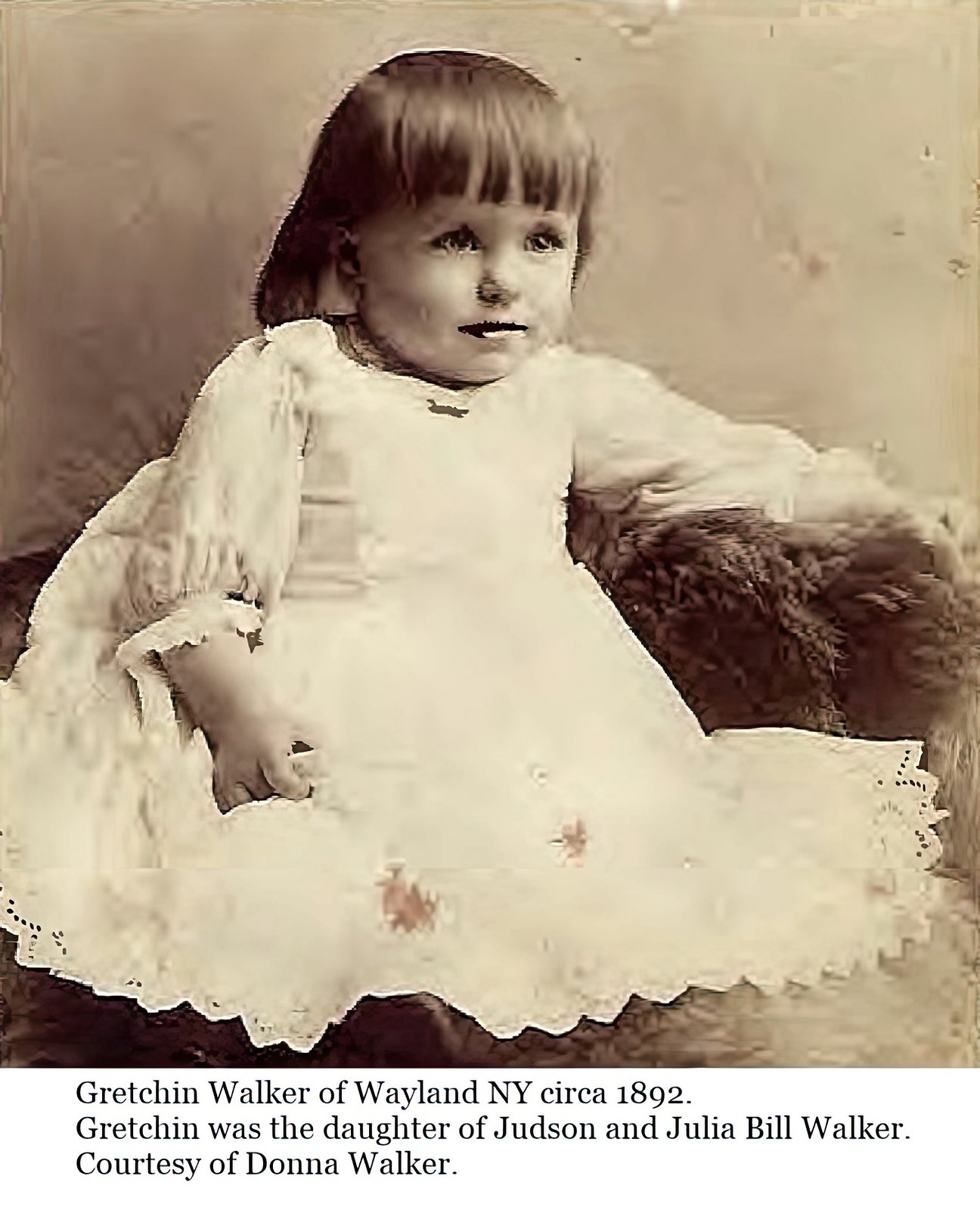This is an old vintage square photograph, sepia-toned, capturing a young girl named Gretchen Walker of Wayland, New York, circa 1892. The image lacks a border and presents a textured brownish background, possibly a wall. Gretchen, appearing to be around two to four years old, has shoulder-length, brown hair with bangs and is wearing an old-fashioned white dress with a ruffled hem and floral patterns. She is positioned facing slightly to the right while looking in that direction with wide-open eyes. Her left hand is resting on something fluffy and brown, likely a pillow or blanket, and her right hand appears clenched. The photograph is slightly blurry due to its age. Below the image, in left-aligned black text on a white background, it reads: "Gretchen Walker of Wayland, New York, circa 1892. Gretchen was the daughter of Judson and Julia Bill Walker, courtesy of Donna Walker."